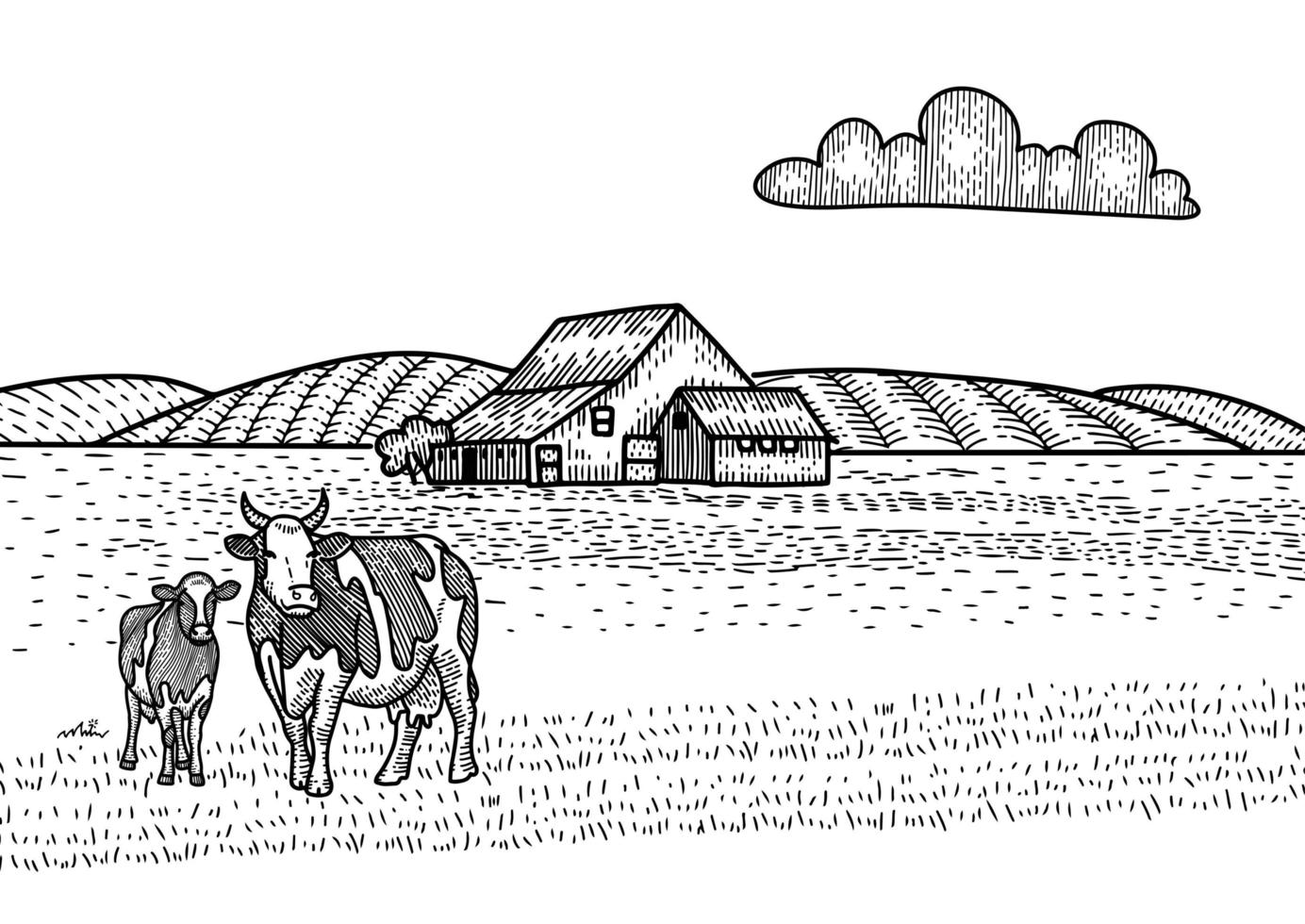This detailed black and white digital illustration features a serene pastoral scene meticulously crafted using only dots and lines. Set against a plain white, borderless background, the rectangular image measures approximately six inches wide and four inches high. Dominating the upper right portion of the image is a whimsical cloud, elongated at about an inch and a half, with a flat bottom and curved, bubbly top, adorned with vertical lines and dots. Below the cloud, rolling hills stretch across, detailed with vertical lines suggesting rows of crops or tilled land.

In the middle ground stands a barn with a steeply sloped roof, accompanied by a smaller structure to its right with its own separate roof. The lower section of the image represents a grassy field, indicated by a pattern of vertical lines and dots. In the foreground, on the lower left side, a horned cow and a smaller, hornless calf — both black and white spotted — add life to the scene. The cow, with an udder, faces left but turns its head towards the viewer, while the calf looks directly ahead. This minimalistic yet richly detailed illustration captures a tranquil rural setting with delightful precision.